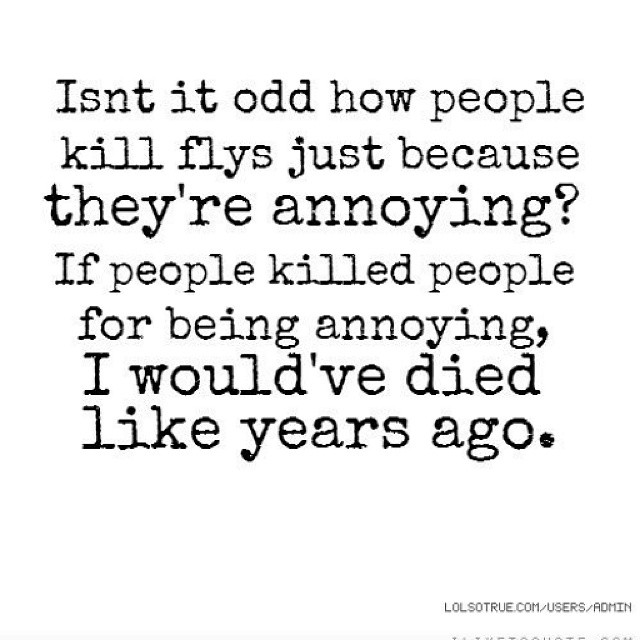This image is a minimalist white square graphic featuring a humorous and slightly philosophical black text, styled to resemble the imprint of a typewriter. The main text, slightly jagged with white spots as if printed by a typewriter with uneven ink distribution, reads: "Isn't it odd how people kill flies just because they're annoying? If people killed people for being annoying, I would have died like years ago." Notably, the word "flies" is misspelled as "flys." In the bottom right corner, there's a small URL that reads "lolsoetrue.com/user/admin," though some of the text is cut off. The stark simplicity of the graphic—with no images or additional decor—makes it a popular choice for sharing on social media platforms like Instagram.